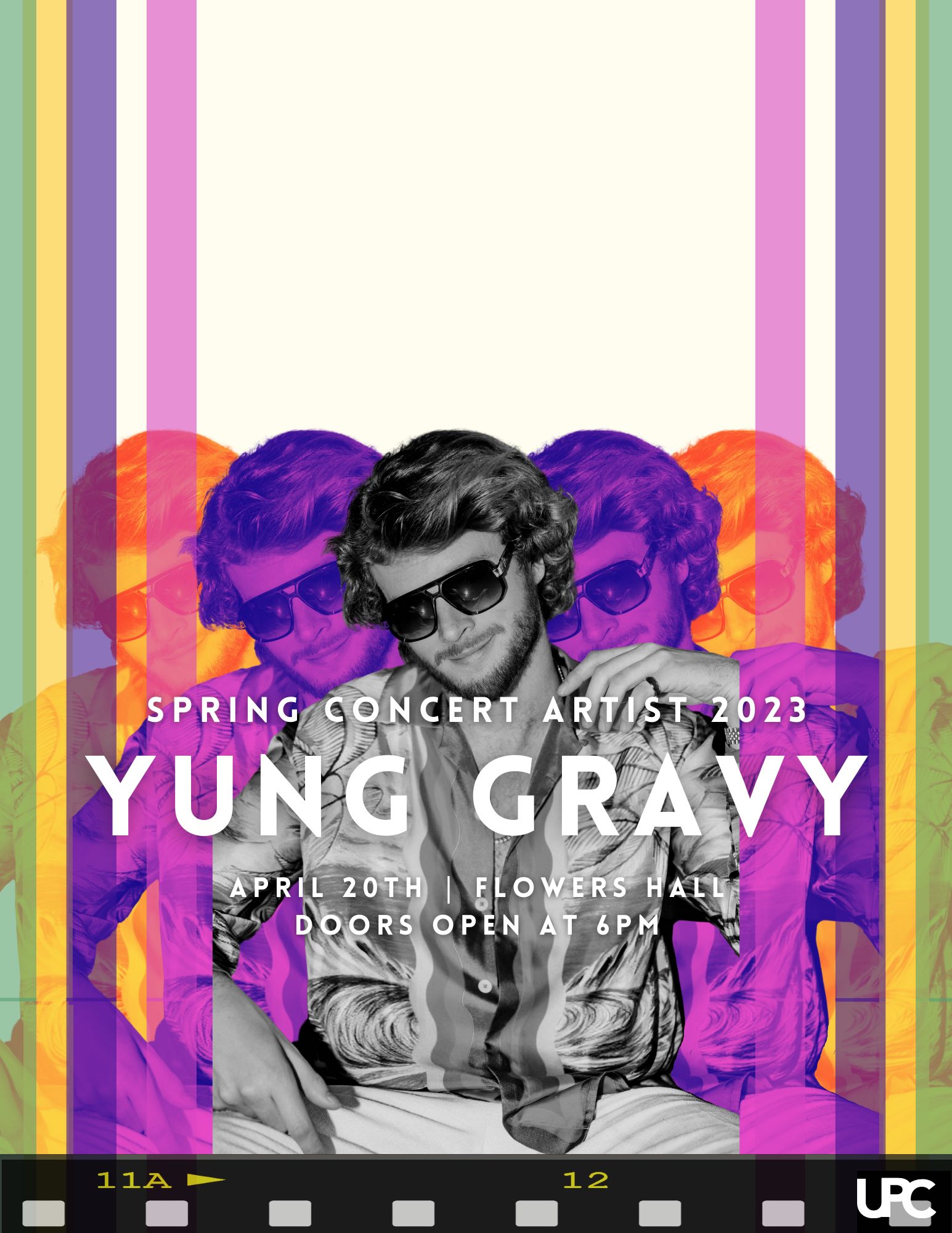The digital poster promotes an upcoming concert, featuring a rich palette of colors. The main background is white, bordered on both the left and right sides by vertical bands of green, yellow, purple, white, and lavender or violet. Dominating the center is an image of the artist, Young Gravy, depicted in a series of five projections. The central portrait is in black and white, flanked by two purple-tinted versions on each side, which are further bordered by two orange-tinted versions at the far edges.

The artist, a young man in his mid to late 20s, has long, wavy light brown hair and wears square sunglasses. He is clad in a shiny, designer shirt with stripes down the front and white pants. His stance is dynamic, with one hand raised over his shoulder and the other resting on his thigh.

The lower part of the poster mimics the style of an old Kodachrome film reel, featuring the numbering "11A" and "12," as well as the UPC logo. In gold, the text on the poster announces the "Spring Concert Artist" event, scheduled for February 2023. Highlighted details include Young Gravy performing on April 20th at Flower Hall, with doors opening at 6 p.m.